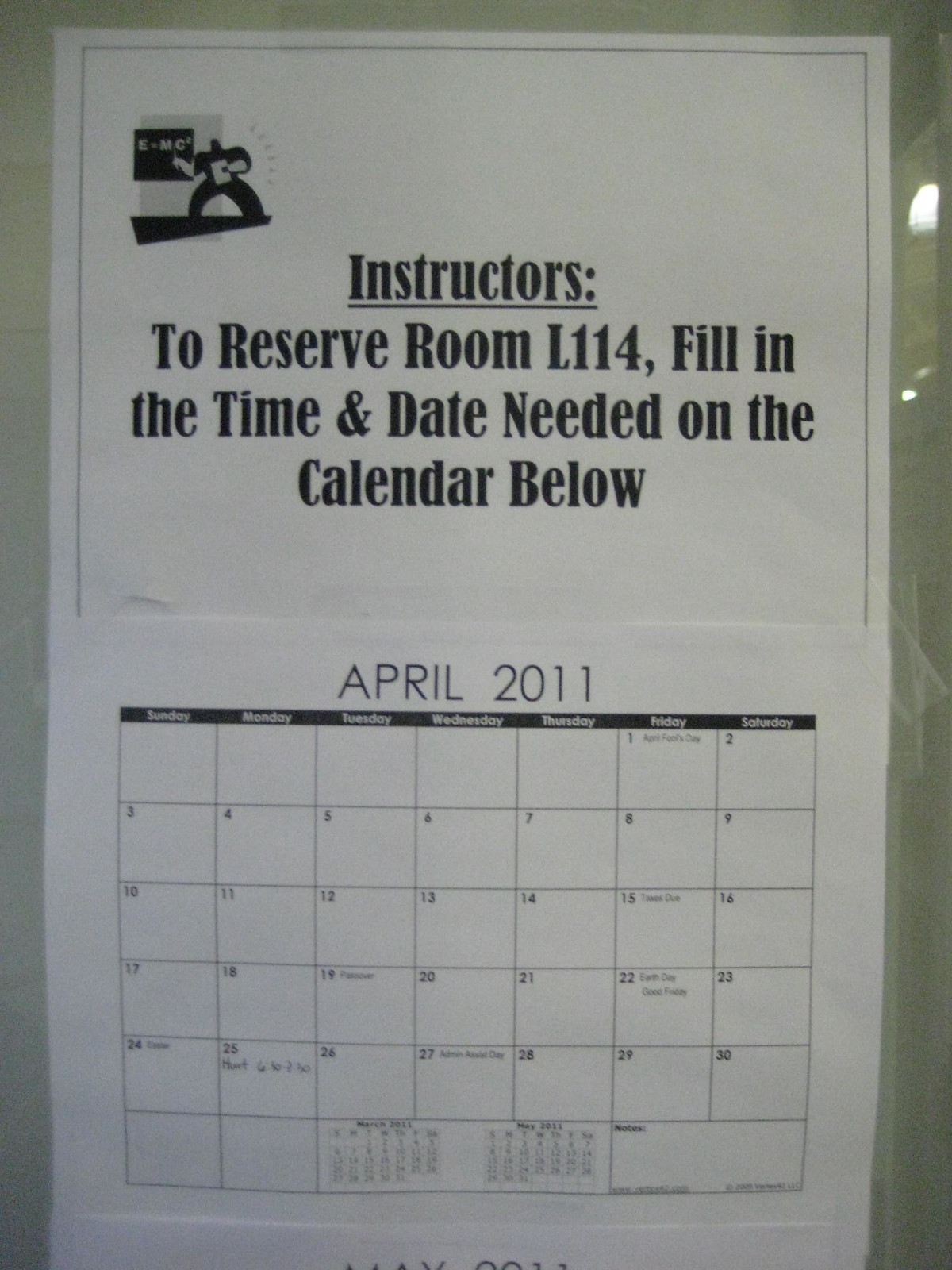The image is of a calendar hanging on a predominantly white or off-white wall. At the top of the calendar, prominently displayed in black text, it reads "Instructors," which is underlined. Below this, an instruction is clearly visible: "To reserve room L114, fill in the time and date needed on the calendar below." The visible calendar is for April 2011, and various entries have been written into some of the day's squares. Notably, on April 25th, there is a reserved slot that reads "6:30," though the second part of the time is slightly unclear. An icon or small image depicting a person writing, accompanied by "E=MC²," is present near the top section. The calendar itself appears to be affixed to the wall with tape. Partially visible below is the beginning of the May 2011 calendar, indicating that multiple months are displayed, though only the edge of May is seen.